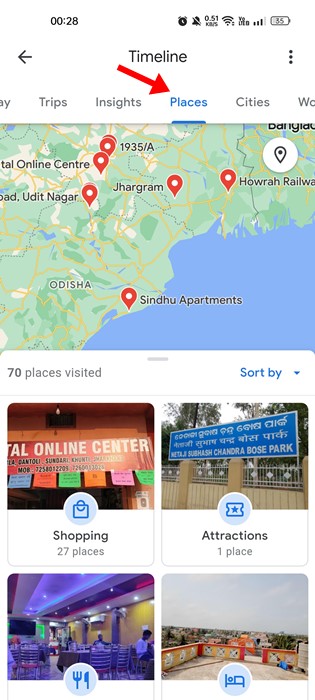The image appears to be a screenshot from a smartphone taken at 00:28, as indicated by the military time shown in the top left corner. The status bar includes various icons: a clock, a muted speaker symbol (denoting that the device is on silent mode), a Wi-Fi indicator, and a battery meter. Directly below the time, there's an arrow pointing left, a central "Timeline" label, and three vertically aligned dots suggesting a menu.

The partially visible interface shows sections for "Trips," and "Places," with the latter being highlighted in blue and underlined. In the main section of the screen is a map displaying several red pins marking specific locations. The map is highly zoomed in, focusing on a geographic region that isn't immediately identifiable.

Key locations marked on the map include:
- Sindhu Apartments, placed near the water.
- Several pins close to Udit Nagar, with a total of four pins close together in this area.

Below the map, the interface indicates that 70 places have been visited, and there is a drop-down menu for sorting. Several categorized sections are visible, albeit partially cut off, including:
- "Shopping" with 27 places listed alongside a relevant image.
- "Attractions" featuring one place.
- A "Food" category that is mostly cut off.
- A section for accommodations, represented with an image of a bed, indicating places to sleep.

Overall, the image captures a detailed view of a location-tracking application interface on a smartphone, including various functional icons, a highlighted "Places" section, map with pinned locations, and categorized lists of visited sites.